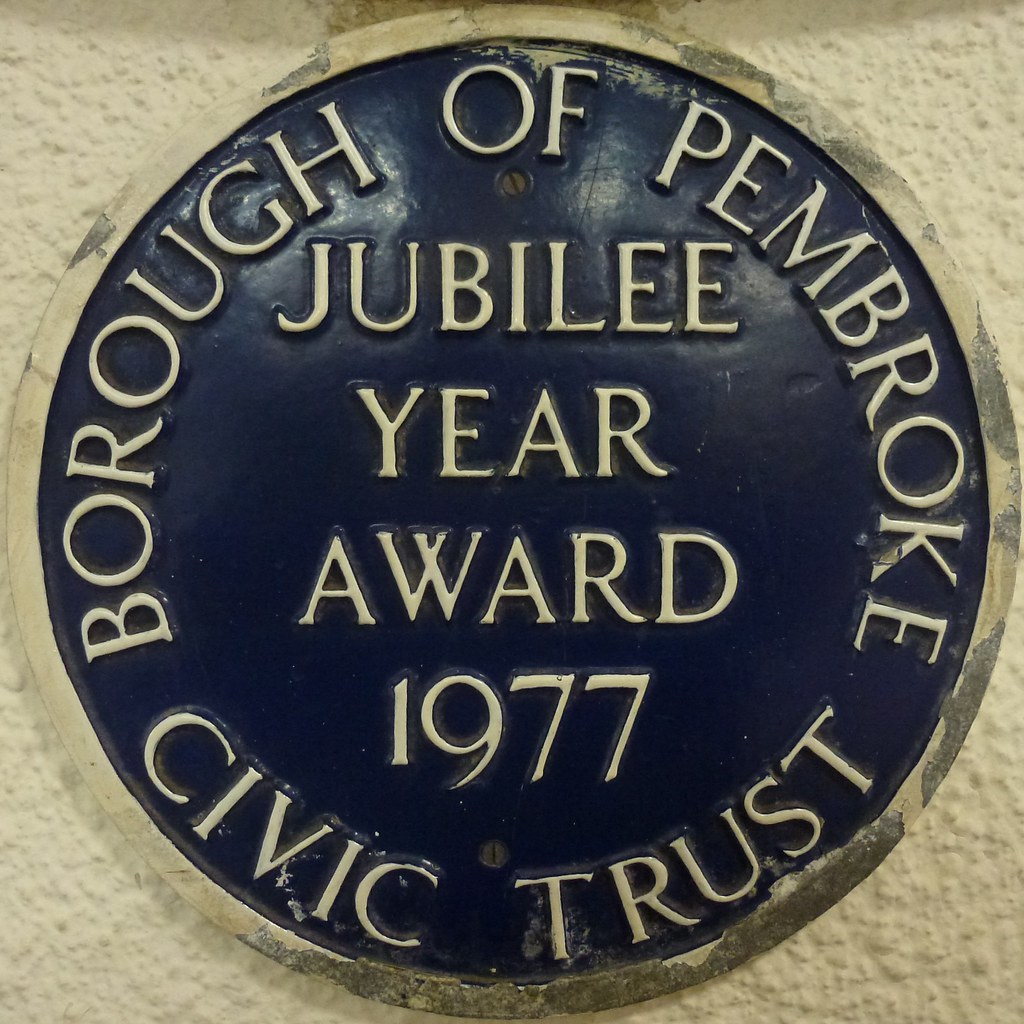The image depicts a circular plaque, a potential emblem or logo, against a textured, painted metal surface. The plaque exhibits signs of age, with peeling off-white paint around its edges, revealing the bare metal underneath. The center of the plaque is a dark navy blue or black, featuring raised, off-white capital letters. The text along the upper curve reads "Borough of Pembroke," while the lower curve spells out "City Civic Trust." Prominently displayed in the center are the words "Jubilee Year Award, 1977." The plaque is screwed into the painted surface, and despite its worn appearance, it distinctly commemorates an award from the Borough of Pembroke's City Civic Trust in 1977.